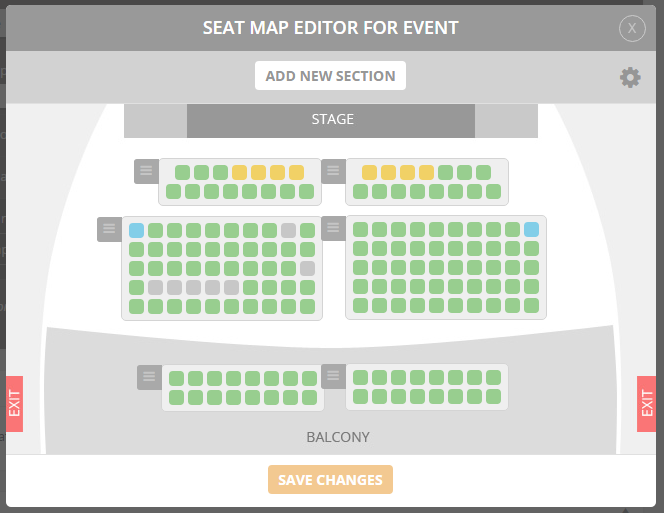This image displays a seating chart typically used for purchasing tickets to a concert, stadium event, or play. The chart appears to represent a small venue. At the top, there's a banner labeled "Seat Map Editor for Event," and just below it, a gray bar indicates the stage area.

The seating layout includes six distinct sections:
- The first two sections on the far left and right each have two rows of seats.
- The middle sections, both left and right, consist of five rows of seats.
- The back two sections, located in the balcony area, also have two rows each.

Most of the seats in the chart are shaded green. In the front row, there are eight seats highlighted in yellow. Within the two middle sections, two seats are marked in blue, which likely signify handicap accessibility. Additionally, there are seven seats depicted in gray throughout the layout. However, there is no legend provided to explain the significance of these colors.